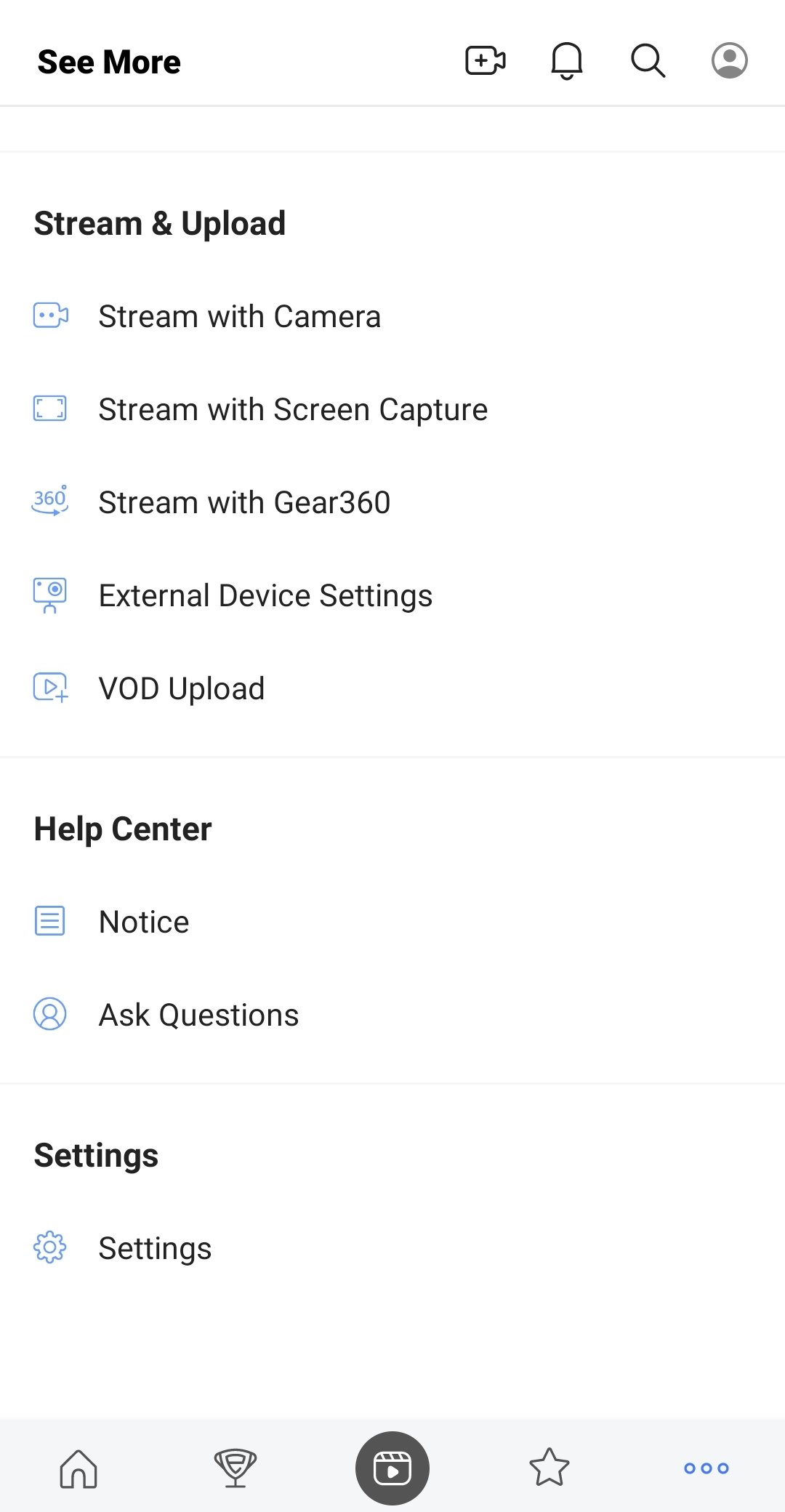The image depicts a screenshot of a mobile device interface titled "Streams and Uploads" at the top. Below the main title, there are several options listed in a structured menu format: "Stream with Camera," "Stream with Screen Capture," "Stream with Gear 360," "External Device Settings," and "VOD Upload." These options suggest functionalities for different streaming and uploading methods available to the user. Further down, there is a secondary menu with tabs labeled "Help Center," "Notice," "Ask Questions," and "Settings," indicating additional resources and customization options. At the bottom of the screen, separated by a light gray horizontal bar, a navigation bar holds buttons for "Home Screen," "Video Clips," and "Favorites." The specific type of mobile device and the platform for which the interface is designed are not identified in the screenshot.